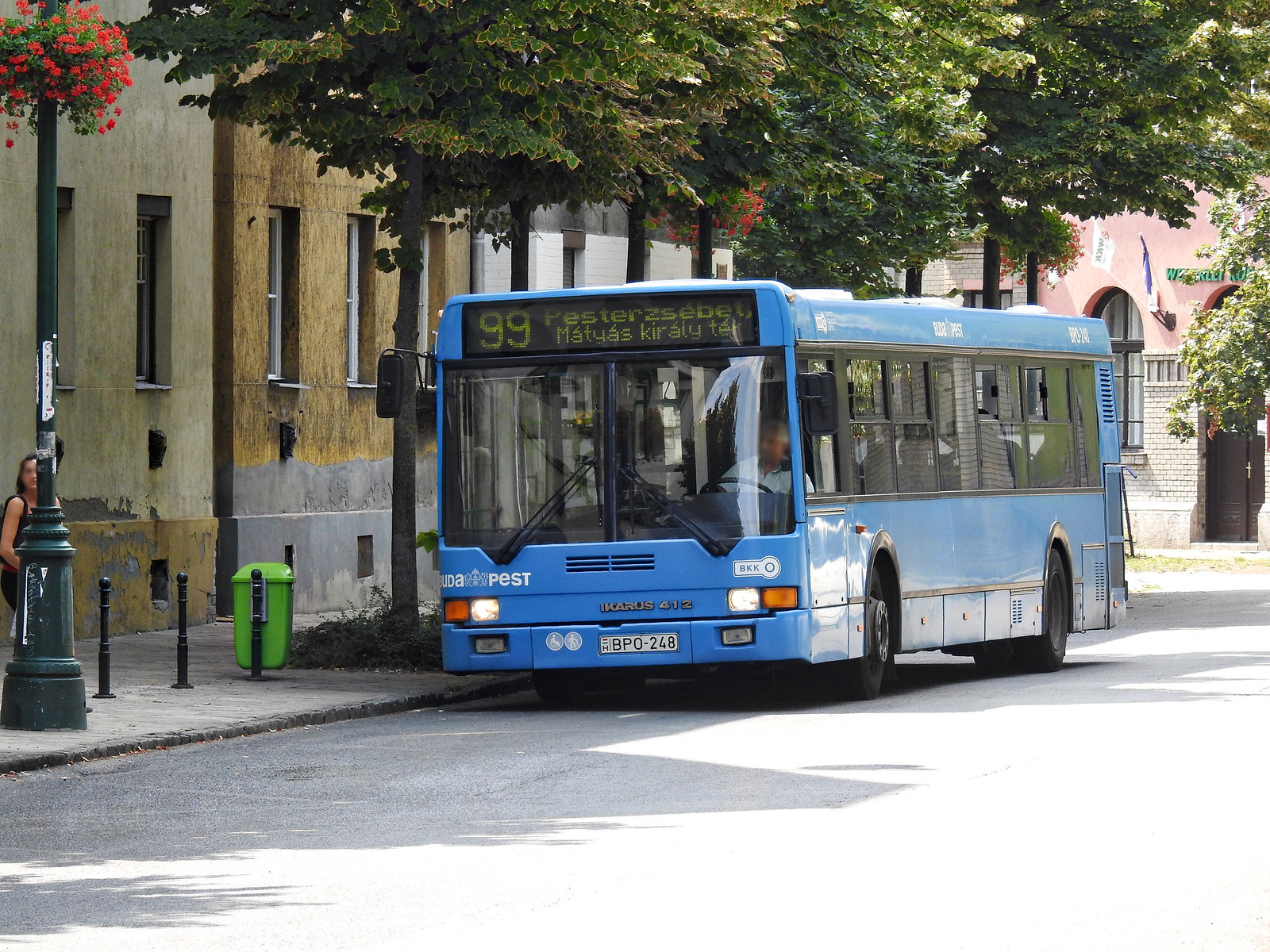In this horizontal, well-lit photograph taken on a sunny day, a blue city bus prominently features in the middle of the scene. The bus, marked with the number 99 in yellow digital font on its front display, also displays some text in an unrecognized foreign language, with words like "PESTER," "ZABET," and "MATYAS KIRALY." The bus, with its large, smoky windows trimmed in black, is parked on a gray asphalt street to the right side of the image. Above the bus, a digital sign in green letters and a white license plate marked "BPO-248" can be seen. 

Flanking the bus on the left is a sidewalk lined with a green trash can and black lampposts. One of these poles features a bouquet of red flowers. A woman with dark hair, wearing a sleeveless shirt, stands behind this pole, partially obscured by it. In the background, there are several city buildings with gray, brown, and white exteriors, featuring set-back windows. The scene also includes small trees with green leaves, reaching above the height of the bus.

Overall, the photo captures a tranquil city moment, with details of urban elements harmoniously blending together under the bright sunlight.